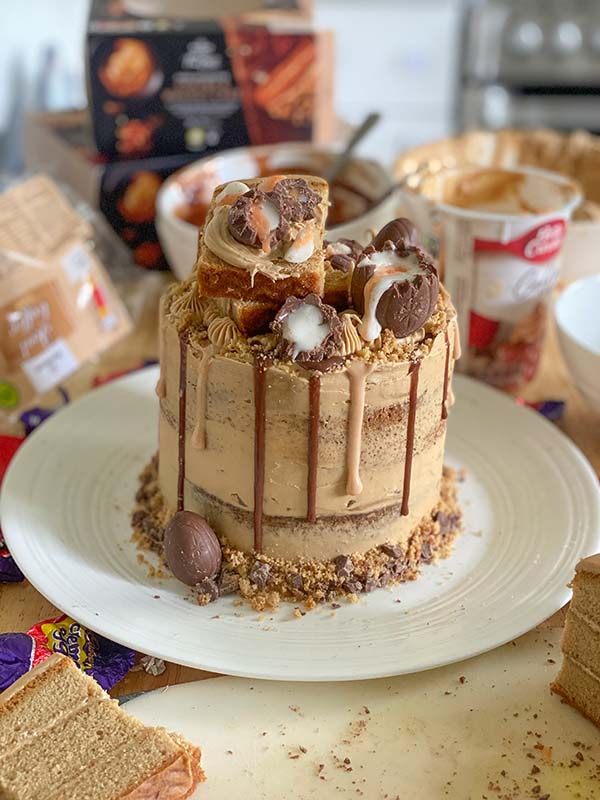This image features a meticulously decorated, multi-layered cake, centrally positioned on a white plate. The cake boasts a light brown color, frosted lightly with caramel-colored icing, accented with both caramel and chocolate frosting that drips down the sides. Crumbled candies and a chocolate egg, resembling a Cadbury egg, adorn the base of the cake. Topping the cake are additional candies and decorative chocolate eggs, with one chocolate egg showing a contrasting white yolk inside. Surrounding the main cake are several slices of a similar cake, neatly arranged. The background showcases Betty Crocker packaging, Cadbury cream egg wrappers, and two bowls of frosting, indicative of the ingredients and effort that went into creating this elaborate dessert. This photograph captures the cake in a kitchen setting, emphasizing the blend of artistry and indulgence in an elegant yet cozy environment.